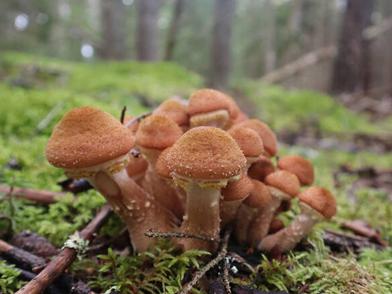The image depicts a densely packed cluster of around 20 unique, brown-colored mushrooms with domed caps adorned with small white speckles and bumpy textures. These fungi are growing together from a shared base in a lush, humid forest setting. The forest floor appears damp, covered in green moss, grasses, undergrowth, and scattered dead twigs and branches, further capturing the moist atmosphere. In the hazy background, there are partially visible tree trunks, with some fallen and others standing, providing a sense of depth and the typical verdant environment of a damp woodland, possibly reminiscent of the UK.